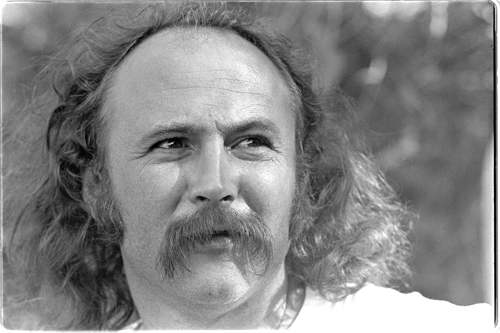This black-and-white photograph features a well-known American musician, David Crosby, likely taken in his late 30s to early 40s. The image captures him with long, brown, curly hair that extends past his shoulders but reveals a significant bald spot on the top of his head, giving him a receding hairline and a prominent forehead. His distinctive, walrus-like mustache is large and hairy, adding a unique character to his friendly and well-natured demeanor. Crosby is wearing a white t-shirt and is looking intently to the right of the camera with a subtle smile on his face. The background is blurred, suggesting he is outdoors, possibly in a backyard with visible tree branches and a hedge. The photograph, with its rounded edges and black border, appears to be a scan from a 35mm film, carefully exposed to create a smooth, soft light on Crosby's face.